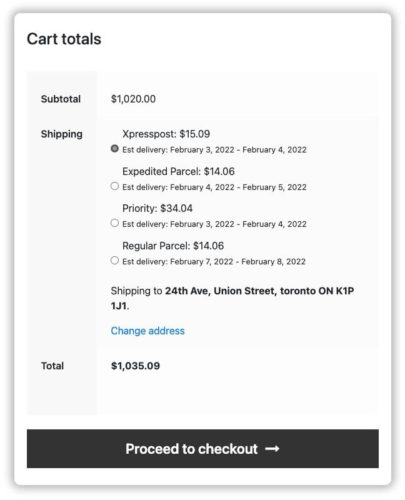The image captures a detailed view of a checkout summary displayed on a white box with black text. At the top of the box, a heading reads "Cart Totals." Listed on the left side are various sections: "Subtotal," "Shipping," and "Total." 

The "Subtotal" section specifies an amount of $1,020. Below this, the "Shipping" section presents multiple shipping options along with their respective costs and estimated delivery dates:
- Express Post: $15.09, estimated delivery between February 3rd, 2022 and February 4th, 2022 (this option is currently highlighted).
- Expedited Parcel: $14.06, estimated delivery between February 4th, 2022 and February 5th, 2022.
- Priority: $34.04, estimated delivery between February 3rd, 2022 and February 4th, 2022.
- Regular Parcel: $14.06, estimated delivery between February 7th, 2022 and February 8th, 2022.

The shipping address is listed as 24th Ave, Union Street, Toronto, ON K1P1J1. Below the address is a blue "Change Address" button. The "Total" section at the bottom of the list shows the amount $1,035.09. 

Finally, a black bar featuring a white "Proceed to Checkout" button is situated at the bottom, allowing the user to complete their order. The total amount reflects the selection of the Express Post shipping option, priced at $15.09.